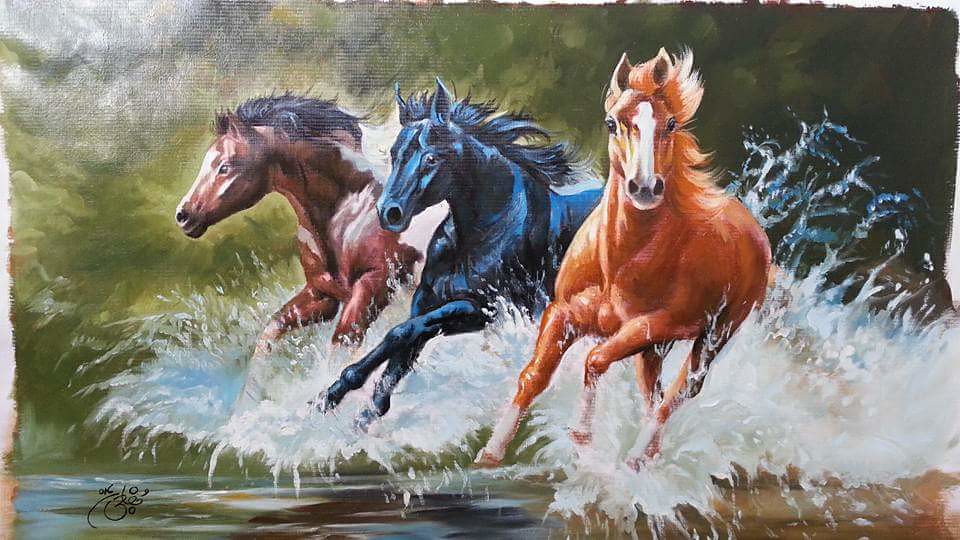This photograph captures an oil-based painting on canvas, depicting three horses galloping dynamically from right to left, slightly towards the viewer. The horses are splashing through a body of water, with the energetic splashes rendered in white with bluish and brownish undertones. The background features a green blur resembling trees, adding depth and context to the scene. 

The horse on the left is a dark brown with a black mane, its nostrils flaring from exertion. The central horse, entirely black and shiny, stands out with its sleek appearance. The horse on the right is a chestnut color, characterized by light brown with white markings on its lower legs and a distinctive white stripe up its nose. This horse’s mane matches its reddish-brown body. The painting's brushstrokes and the slight reflection on the top left, possibly from a camera flash or artificial light, hint at the texture and medium of the artwork, enhancing the vivid and lively portrayal of the horses splashing through water.